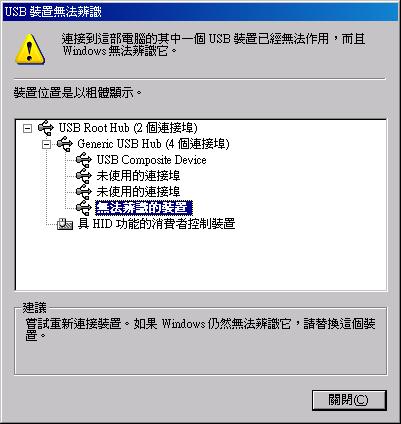The image portrays a screenshot featuring a gray background with a navy blue banner at the top. On the far left of this banner, the text "USB" is prominently displayed in English, followed by characters that resemble Chinese, Japanese, or Korean script. Below this banner, towards the top-left side, there is a large yellow triangle containing a black exclamation point. The rest of the screen is filled with non-English characters, but the word "windows" can be deciphered among them. The gray background section encompasses a white box that stands out at the center. Inside this white box, the top line reads "USB Root Hub," followed by "Generic USB Hub" on the second line, "USB Composite Device" on the third line, and "HID" appearing further down. This detailed image seems to show a dialog box or system utility related to USB device management, part of an interface that includes Asian language text.